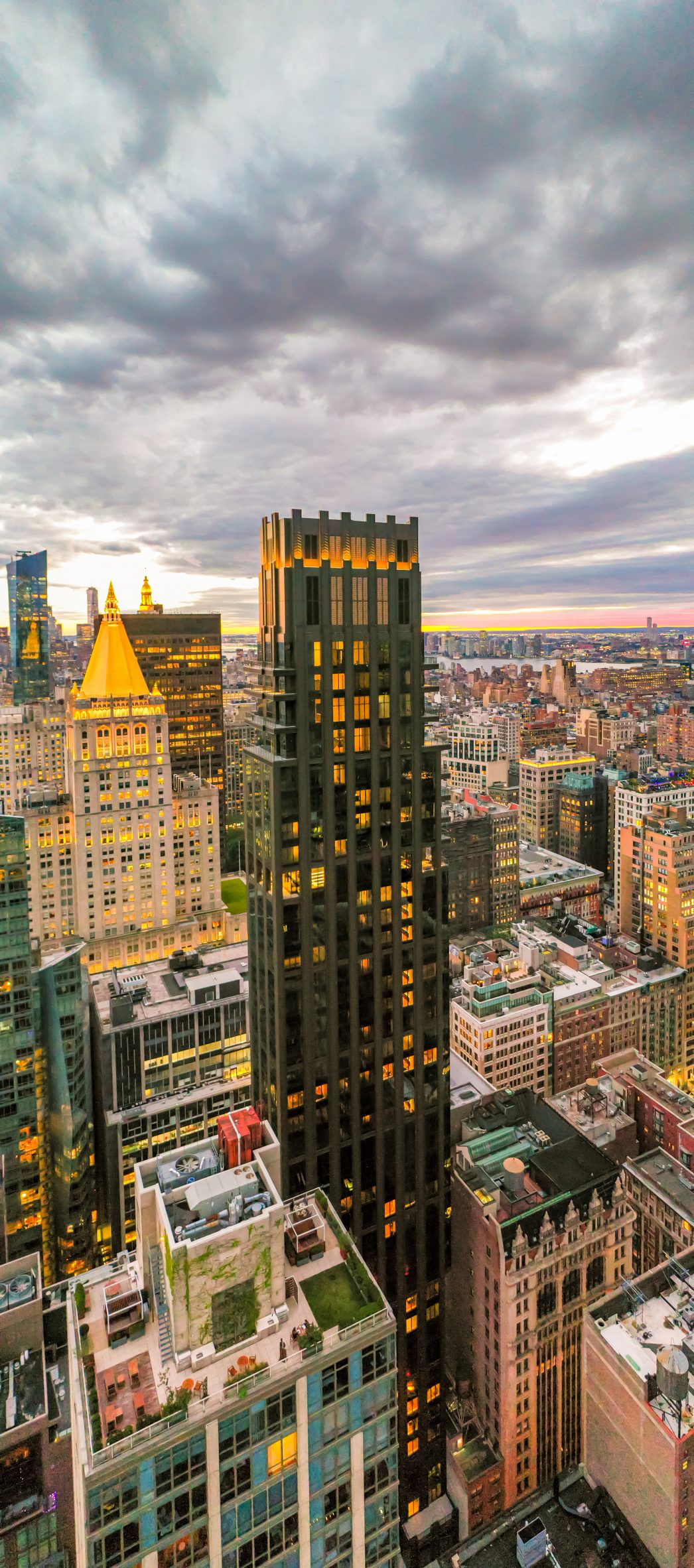The image is a painting of a metropolitan cityscape captured from an aerial viewpoint. It features a gloomy, gray sky thick with stormy clouds, faintly illuminated by a gradient sunset with hints of pink and yellow. Dominating the center foreground is a slender, multi-storied black skyscraper, its interior warmly glowing with orange lights. Surrounding this central skyscraper are various buildings of differing heights, colors, and architectural styles, ranging from modern glass structures to more eclectic designs. Among these neighboring buildings, one has a distinctive red structure atop it. The scene is detailed with clean, black roads weaving through the cityscape, adding to the orderly yet bustling urban atmosphere.